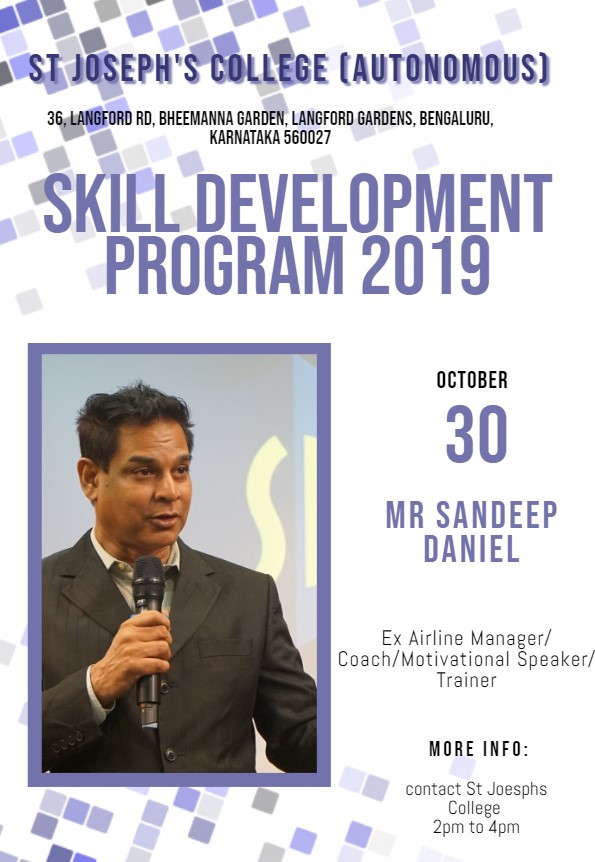The image is a detailed promotional poster for an event at St. Joseph's College (Autonomous) located at 36 Langford Road, Bihamana Garden, Langford Gardens, Bengaluru, Karnataka, 560027. The header reads "Skill Development Program 2019" in prominent blue letters on a white background, with the date "October 30" noted beneath. Featured on the left-hand side of the poster is a photograph of Mr. Sandeep Daniel, who is identified as an ex-airline manager, coach, motivational speaker, and trainer. Mr. Daniel, captured mid-speech, is wearing a gray suit with a light brown shirt and is holding a microphone close to his mouth. The colors used in the poster include purple, gray, white, black, yellow, tan, and brown. Additional details on the right side of the image indicate the event's time from 2 p.m. to 4 p.m., with further contact information available through St. Joseph's College. The layout clearly emphasizes the important event information and includes a vivid picture of the speaker, making it both informative and visually engaging.